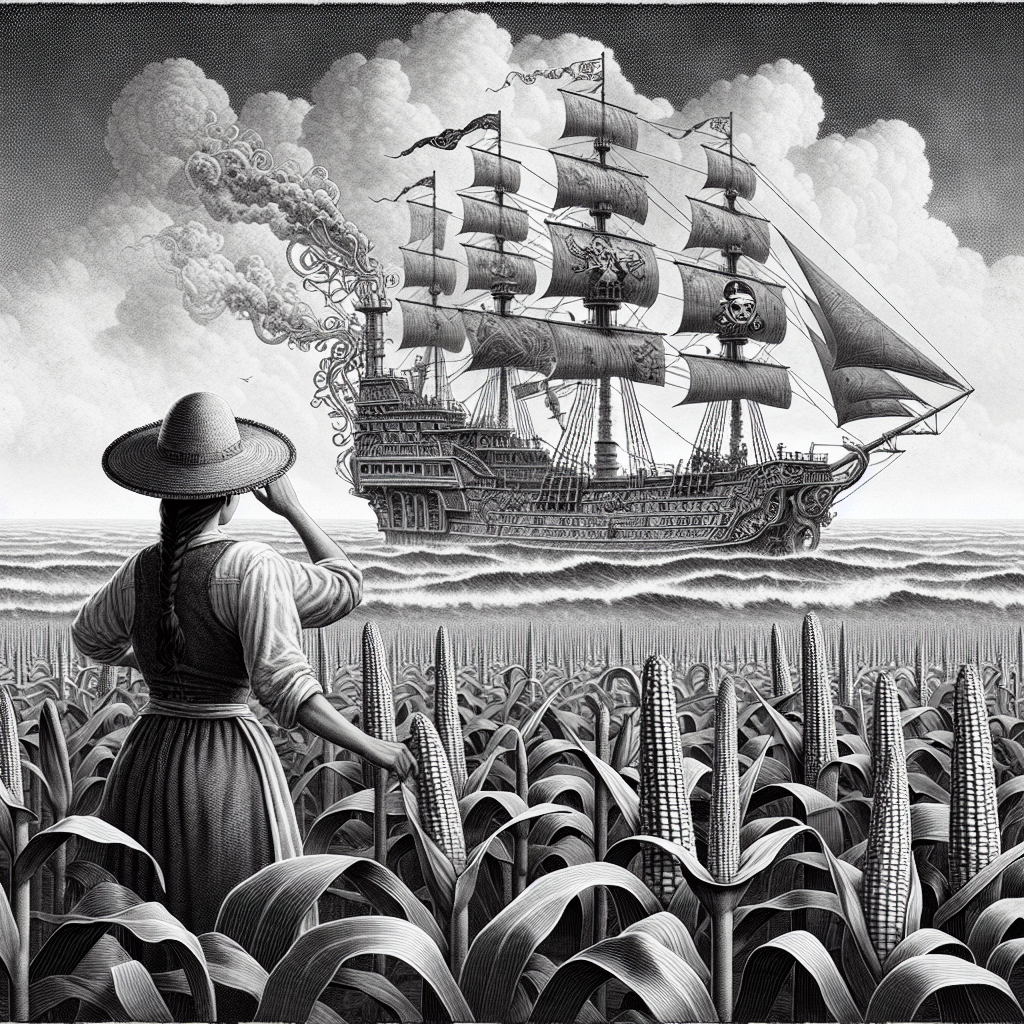This hyper-realistic, black-and-white pencil drawing presents a surreal scene of a young girl or woman standing in an infinite cornfield. She wears a wide-brimmed sun hat and has a long dark braid. In a bizarre twist, she has three arms; one left arm resting at her waist, one right arm holding an ear of corn, and the other right arm touching her face. She gazes out toward the distance where a colossal pirate ship with numerous sails and several pirate flags sails on the ocean amidst high waves. Smoke, eerily resembling octopus tentacles, billows from a steam engine at the back of the ship. The image captures intricate details in black, white, and gray shades, emphasizing a mysterious and finely detailed monochromatic scene.